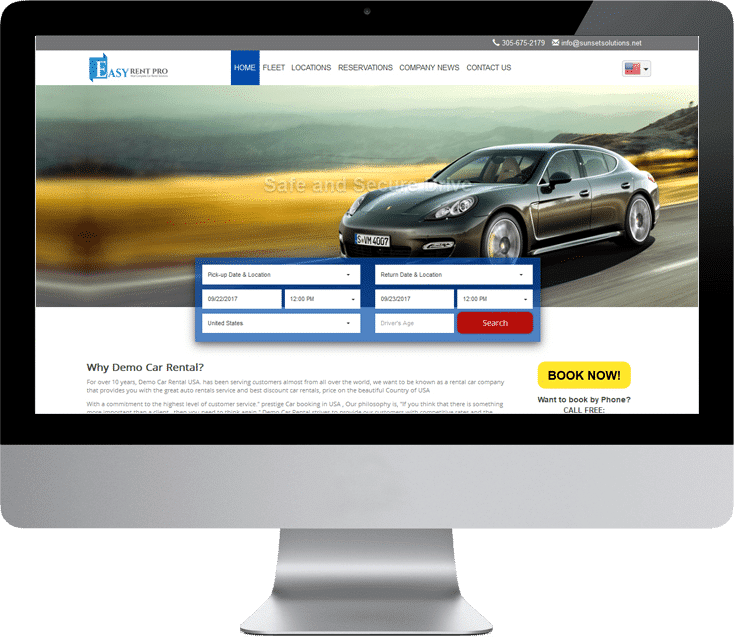A sleek computer monitor is shown with a distinctive gray bottom and a sturdy gray stand positioned centrally to elevate the screen. The monitor features a black border framing the display area. At the top of the screen, a small, dark gray border contains a phone number and an email address, though the details are too minute to discern clearly.

Below this, a white border houses the logo "EZ Rent Pro," with "EZ" in blue and "Rent Pro" in black. To the right of the logo, there is a navigation menu displaying options for "Home," "Fleet," "Location," "Reservation," "Company News," and "Contact Us." Additionally, a language drop-down menu, showing the American flag, suggests language selection capabilities.

Dominating the center of the display is a photograph of a sprawling, yellowish-brown grassy area, with distant, fog-shrouded mountains creating a picturesque yet hazy backdrop. A sleek, black sports car is captured driving towards the left side of the scene, adding a dynamic element to the tranquil landscape.

At the bottom of the screen is a blue box designed for user interaction, featuring fields for inputting information, thus making the interface user-friendly and functional.